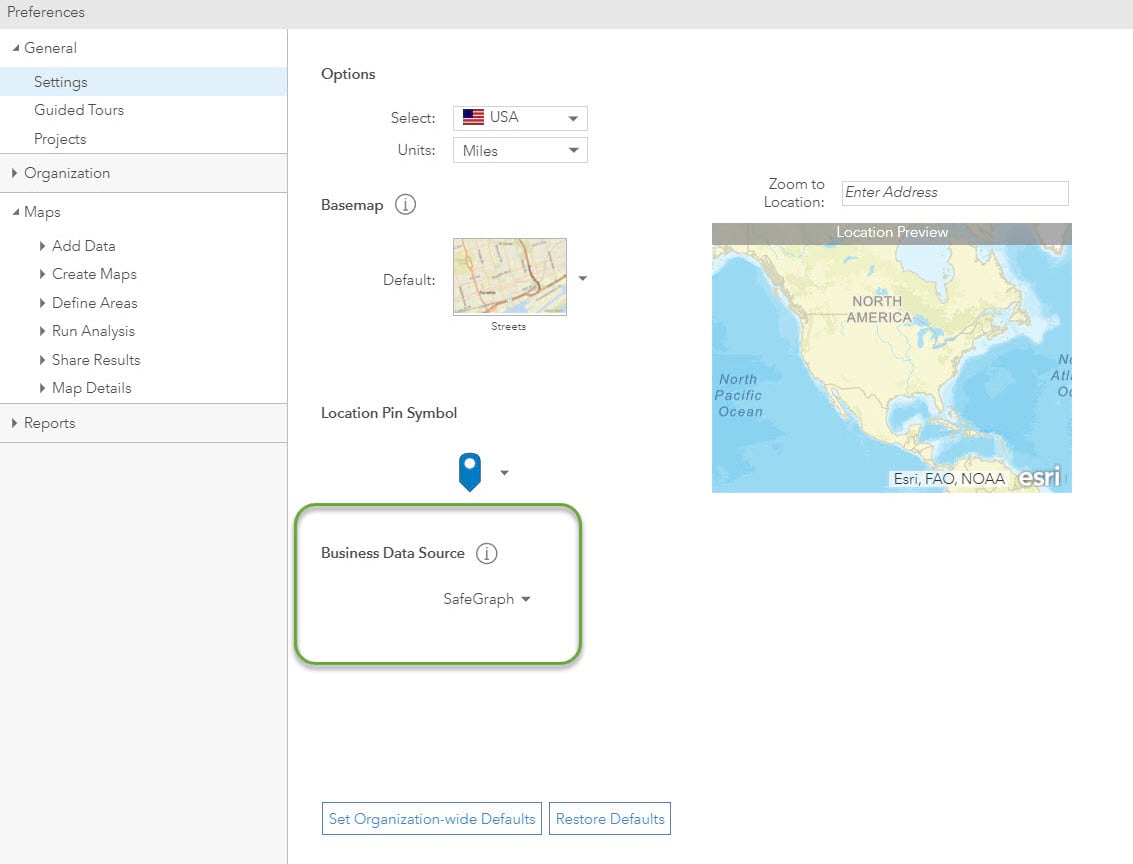Here is the cleaned-up and detailed descriptive caption for the image:

---

**Screenshot Description:**

The screenshot captures a web page interface with a two-pane layout. The top of the page features a gray bar with the headings "Preferences" and "Black."

**Left Pane:**

- A vertical menu with multiple categories and options:
  - **General** (collapsed)
  - **Settings** (highlighted in blue)
  - **Guided Tours**
  - **Projects**
  - **Organization** (expanded, revealing further options)
  - **Maps**
  - **Add Data**
  - **Create Maps**
  - **Define Areas**
  - **Run Analysis**
  - **Share Results**
  - **Map Details**
  - **Reports**

**Right Pane:**

- Predominantly white background area:
  - At the top-left corner, there is a heading: **Options**
  - Below this, there are two drop-down menus:
    - **Select:** Currently set to "USA," accompanied by an icon of the American flag.
    - **Units:** Currently set to "Miles."

  - Below the drop-down menus:
    - A heading: **Base Map** with a small map thumbnail labeled "Default" and "Streets."
    - A label: **Locate Pin Symbol** followed by a green square containing the text "Business Data Source."
    - Underneath the green square: **SafeGraph** (likely indicating the data source).

  - To the right side:
    - A picture element with text: **Zoom to Location** and a search bar labeled "Enter Address."
    - A visible map displaying parts of North America, including the North Pacific Ocean and the Atlantic Ocean.

  - At the bottom of the right pane:
    - Two options: **Set Organization-Wide Defaults** and **Restore Defaults.**

---

This detailed description outlines the structure and contents of the web page, providing clear context for each element depicted in the screenshot.